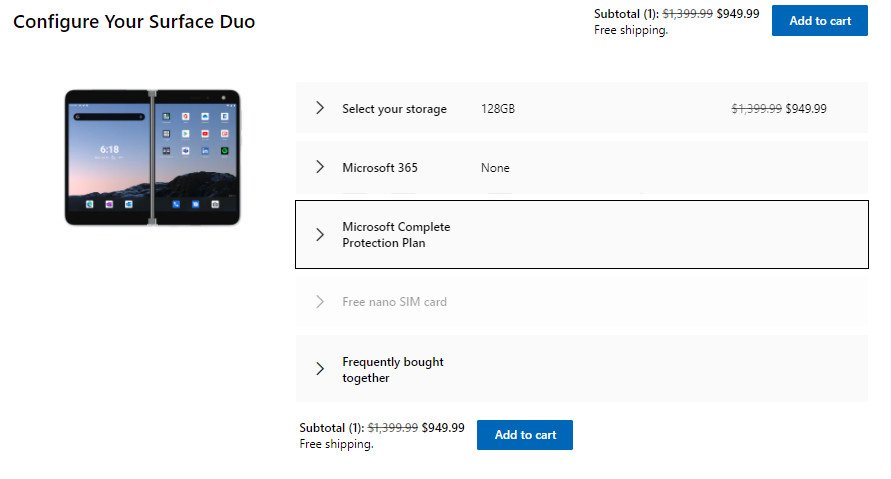This image is a landscape-mode screenshot of a web page detailing the configuration and purchase options for the Microsoft Surface Duo. 

### Top Section:
- **Top Left Corner:** In bold text, it says "Configure your Surface Duo".
- **Top Right Corner:** The text reads "Subtotal: 1". An original price of $1,399.99 is scratched out and replaced with a bolded $949.99. Below this, it notes "Free shipping" and features a prominent blue "Add to cart" button. 

### Main Section:
**Left Half:**
- There is an image of the Surface Duo, illustrating its dual-screen design that folds together. The device's display spans both the left and right sections, displaying various app icons, enhancing the visual appeal. 

**Right Half:**
- The first row, adjacent to the left-side image of the device, includes text prompting users to "Select your storage." The option chosen here is 128 GB, aligning with the $949.99 price.
- Below this, there are details about "Microsoft 365" with the selection marked as "None".
- The next section highlights the "Microsoft Complete Protection Plan" with a darker highlight and a black box around it.
- It also mentions a "Free nano SIM card," though the text is faint, indicating unavailability.
- There is an interactive option labeled "Frequently bought together," allowing users to explore additional related products.
- At the very bottom right corner, the same pricing and "Add to cart" button from the top are repeated: $949.99 and "Add to cart."

This detailed configuration and checkout page aims to provide all essential information at a glance while allowing easy customization and purchase of the Surface Duo.